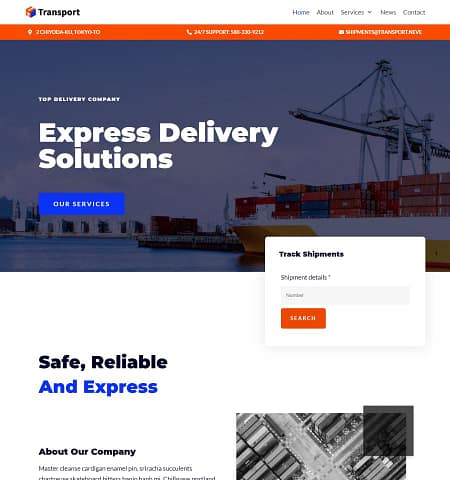The image showcases a website named "Transport." At the top of the page, there is a navigation bar featuring menu items: Home, About, Services, News, and Contact. Dominating the upper section is a large, slightly hazy picture with undertones of dark blue and purple, suggesting a sky at either dusk or dawn. The image includes a body of water with a cargo ship positioned on the right side. 

On the left side of this picture, bold white text declares, "Top Delivery Company, Express Delivery Solutions." Just beneath this text is a rectangular blue button labeled "Our Services" in white. Adjacent to these elements, situated on the right side of the image, is a white box for tracking shipments. It prompts users with the text “Track Shipments” followed by “Shipment Details” and an asterisk. Inside the box, there is a space designed for entering tracking numbers and a reddish-orange search button. 

Below this main area, to the bottom left, a slogan reads: "Safe, Reliable and Express," with "Safe" and "Reliable" in nearly black text and "Express" in dark blue. Further down, there is text beginning with "About Our Company," followed by "Master Cleanse Cardigan Enamel Pins," along with additional, illegible words. To the right of this text, a contrasting black-and-white image is placed, adding a classic touch to the modern webpage design.